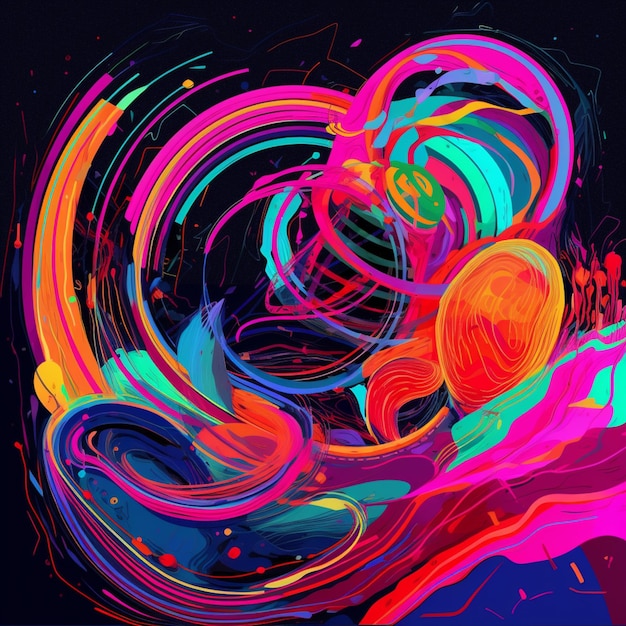This abstract painting in the synthwave style features a dynamic array of bright neon colors—predominantly pink, blue, purple, yellow, orange, and neon green—on a black background. The painting is distinguished by a central arrangement of concentric circles and swirling patterns. The top right corner showcases another set of circles or curved lines in similar vibrant hues. A few speckles of paint punctuate the composition. In the bottom left corner, a roughly kidney bean-shaped area of darker blue paint is smeared with pink and orange swirls extending from its top, intersecting with the other circles. An orange oval, reminiscent of an egg yolk, prominently occupies the middle right side. In the bottom right corner, thicker smears of light blue, pink, and purple paint form an intricate design, completing the psychedelic, wavy, and convergent element of the artwork.